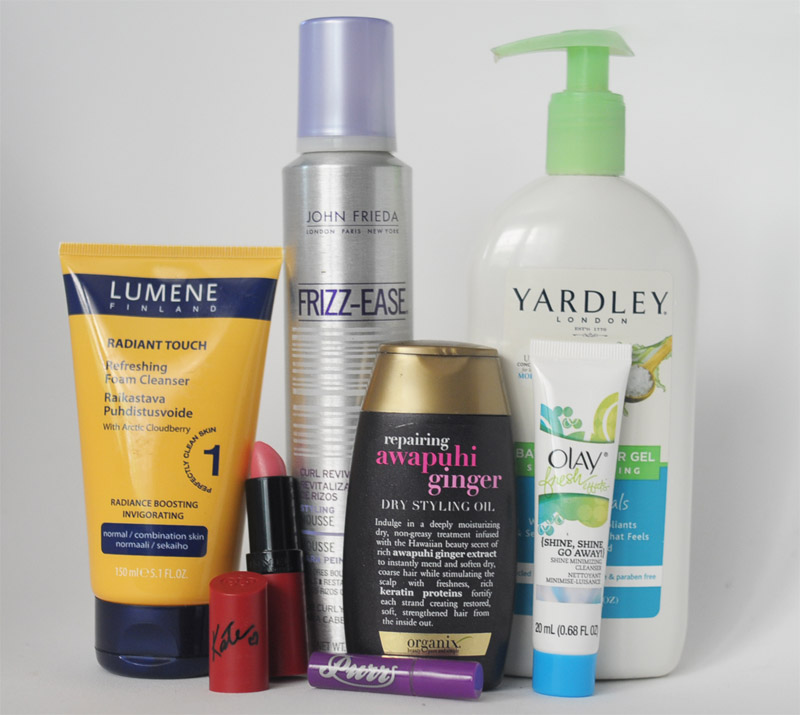The photo showcases an assortment of beauty products, each serving a distinct purpose. Prominently featured is a yellow tube labeled "Lumene," a product from Finland identified as the "Radiant Touch Refreshing Foam Cleanser," designed for facial use. Next to it stands a silver tube from John Frieda, named "Frizz Ease," which appears to be a type of hairspray. Adjacent to these is a white container from Yardley, London, equipped with a green pump top; this container holds a gel, though its specific label is partially obscured. In front of the Yardley product is a compact white tube from Olay, marked "Fresh Effects Shine, Shine Go Away," distinguishable by its blue lid. Lastly, there is a squat black and gold container named "Repairing Awapuhi Ginger Dry Styling Oil," completing the diverse range of beauty essentials depicted in the image.